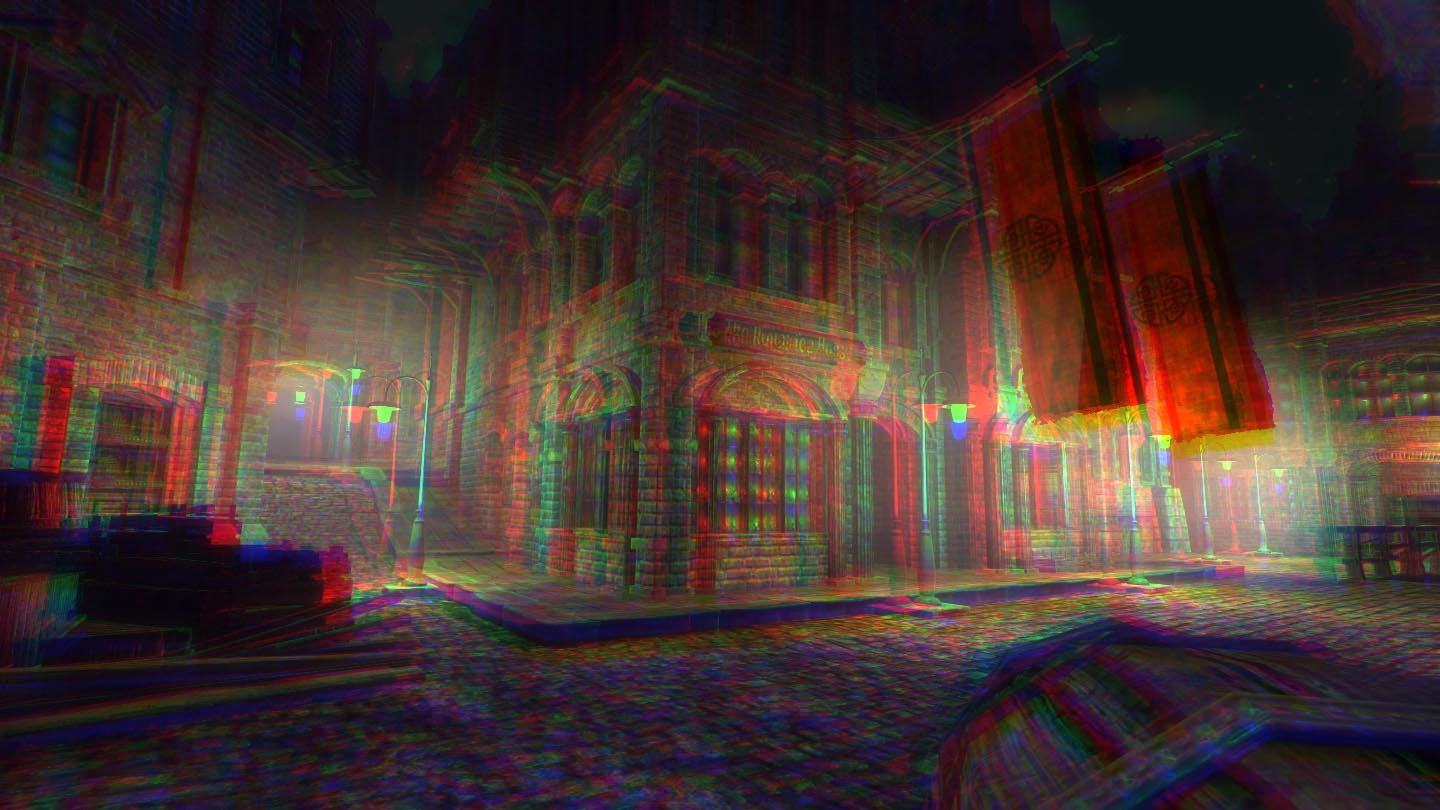This 3D rendering, likely from a video game or art program, depicts a distorted, rainbow-colored European-like city scene. The rendering is heavily stylized with a gradient effect creating multiple colorful afterimages. The cobblestone street stretches from the foreground, leading left through an archway and right along additional streets, flanked by multi-story stone townhouses. Notably, there is a 3D barrel with a silver band lying on its side in the bottom right corner. The main central building, appearing as a storefront with a sign and awning, is crafted from brick and adorned with hues of red, yellow, and blue. Above this building, a large red flag hangs prominently. In the upper right-hand corner, two red flags with black stripes and yellow accents hang as well. A small alley to the left reveals hanging green and blue lamps. The skies above transition in shades of dark and light gray, providing a moody ambiance to the setting. Patterns of yellow and blue mosaic the windows, enhancing the surreal visual effect, while silver lampposts, appearing bluish, illuminate the scene, casting yellow and blue light on the brick-like street and gray sidewalk.